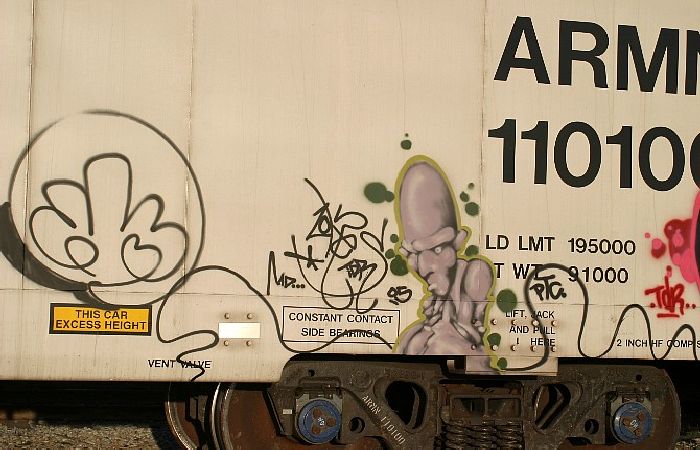The photographic image depicts an outdoor daytime scene of a freight train boxcar, primarily cream-colored and extensively tagged with graffiti. The boxcar features bold black lettering prominently displaying "RM 11010," followed by additional text including "LD LMT 195000" and "WT 91000." On the right side, there is detailed print indicating specific compliance and safety information, reading "This car exceeds height constant contact side bearings FT and Lift jack and pole here two inches too high in CH HFC OMP."

The lower section of the car is heavily adorned with graffiti. On the left side, a prominent logo resembling a raised middle finger is flanked by abstract squiggles and letters that partially read "M," "T," and "PTG." Among the vivid illustrations, there is a notable depiction of a distorted alien figure characterized by a gray elongated head, ridged eyebrows, overhanging small eyes, and a pouting expression, with green splotches accentuating the surrounding area. The image also captures a fragment of the wheels and the truck underneath, labeled "AR I N 110 100."